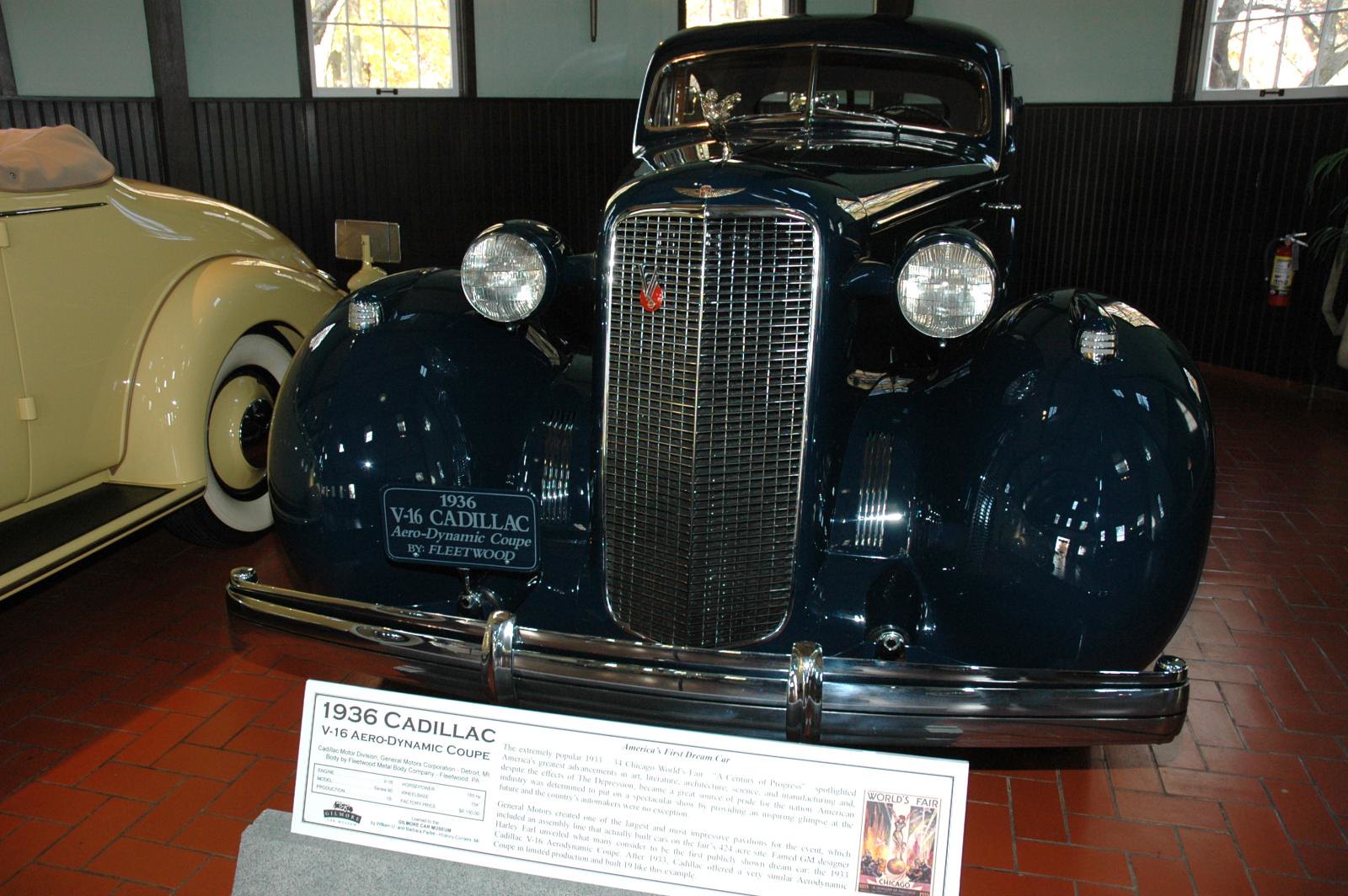The image is a horizontal, rectangular photograph featuring a meticulously restored 1936 V16 Cadillac Aerodynamic Coupe by Fleetwood, on display in a museum with a historic ambiance. The car, gleaming and polished to perfection, stands prominently on a red brick floor. Its headlights and silver grille are in impeccable condition, reflecting the high level of care it has received. A sign mounted on the front of the car reads "1936 V16 Cadillac," with an additional detailed sign placed in front that describes the car's significance as "America's first dream car." This car, introduced at the World's Fair in Chicago, boasts large fenders, a small windshield area, and a distinctive hood ornament. The wall behind the car is painted green with a wooden wainscot, contributing to the museum's vintage feel. Adjacent to the black Cadillac, a portion of a yellow antique car of a similar style is visible, suggesting the presence of other classic vehicles in the museum. Windows along the back wall hint at the building's vast collection of historic automobiles.